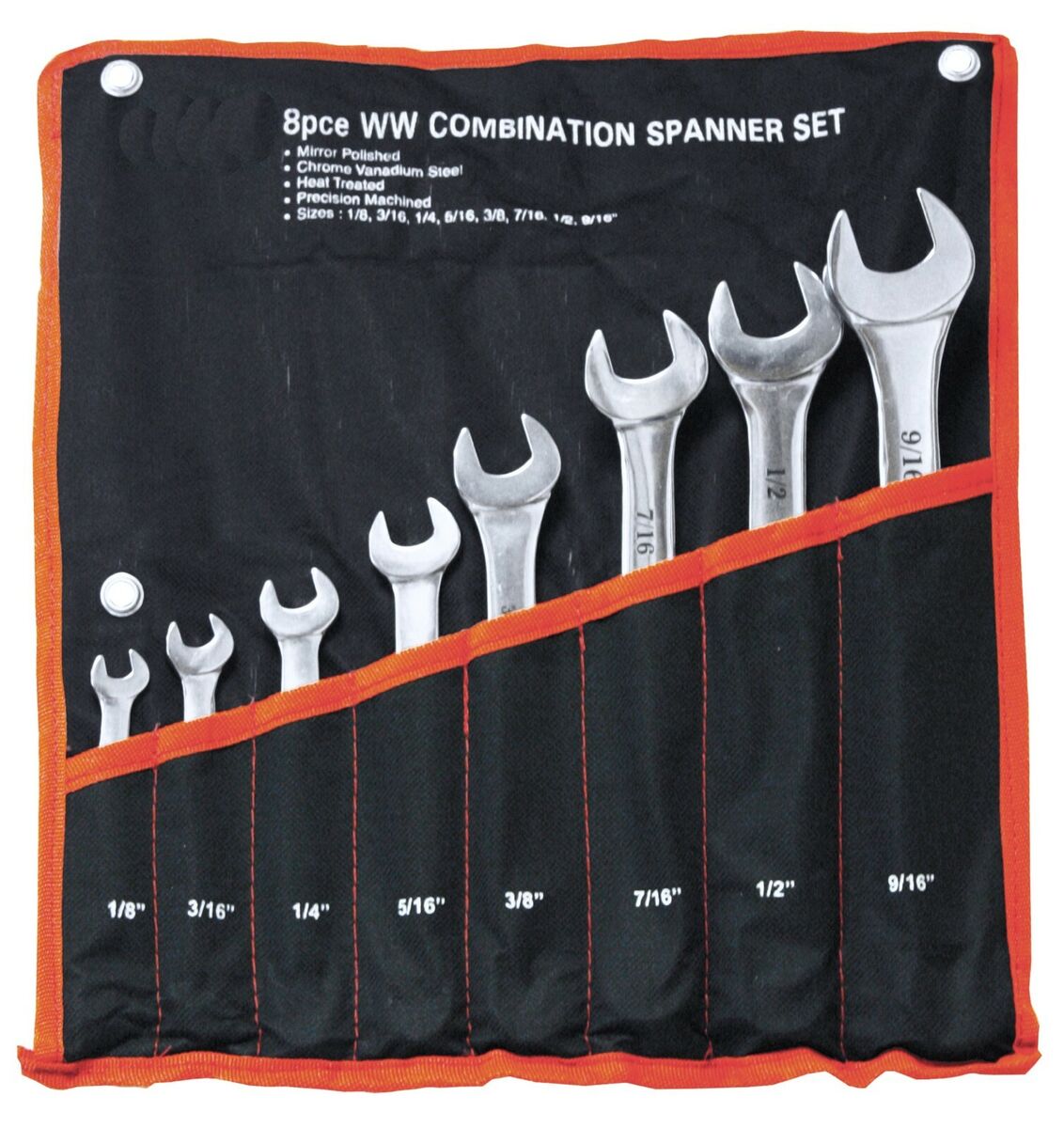This image depicts an eight-piece combination wrench set organized in a black fabric carrying case with a red border. The set consists of individual pockets, each separated by red stitching, holding wrenches of various sizes, including 1/8", 3/16", 1/4", 5/16", 3/8", 7/16", 1/2", and 9/16". Every pocket is clearly labeled with its respective size in white text. The wrenches are made of shiny, mirror-polished chrome vanadium steel, known for its durability and high quality. Printed on the top of the fabric in bold white text is "8 PCE WW Combination Spanner Set", followed by bullet points mentioning the key features: mirror-polished chrome vanadium steel, heat-treated, precision-machined, and the included sizes. The overall presentation suggests a sturdy and well-organized set, ready for use or transport.